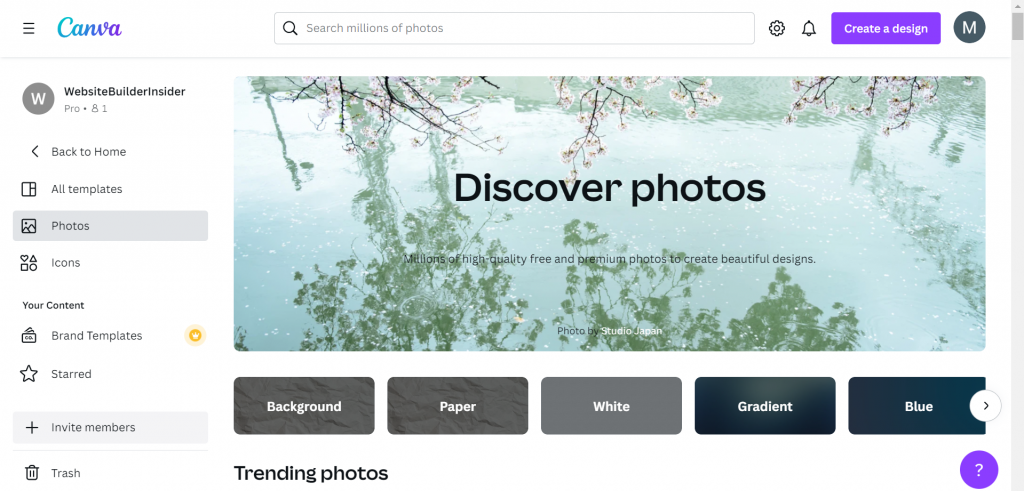Screenshot of Canva's Webpage

The screenshot showcases the Canva web interface in detail. The recognizable Canva logo is prominently displayed in the upper left-hand corner. On the opposite side, in the upper right-hand corner, a purple rectangle featuring the text "Create a Design" invites users to start a new project. 

The left-hand side of the page is occupied by a vertical menu with several navigational options starting from the top: Website Builder Insider Pro 8.1, Back to Home, All Templates, Photos, Icons, Your Content, Brand Templates, Starred, Invite Members, and Trash.

Central to the page is a striking, long rectangular photograph. The image exudes tranquility, featuring a watery surface in a light, almost turquoise blue hue. Delicate cherry blossom branches stretch horizontally across the top of the photograph, while reflections of green leaves elegantly adorn the bottom half of the image.

Overlaying the center of the image is a text banner stating: "Discover Photos, Millions of High-Quality Free and Premium Photos to Create Beautiful Designs." This serves as an inviting prompt for users to explore Canva's extensive photo library.

Beneath the central image, a horizontal menu displays options for various background choices labeled as follows: Background Paper, White, Gradient, and Blue.

This detailed layout of Canva’s interface highlights its user-friendly design and abundant resources for creating visually stunning designs.